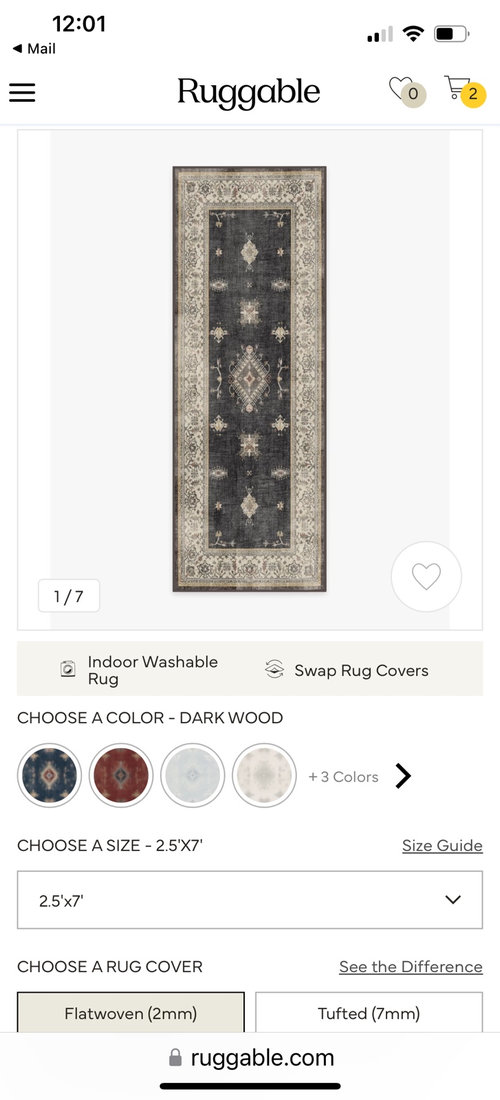**Ruggable Web Page Display on User's Phone**

The screenshot captures a moment on a user's phone while browsing the Ruggable website (ruggable.com) at precisely 12:01. The user had just navigated from their mail, indicated by the back arrow for returning to mail. The phone's status bar shows about 60% battery life and a couple of bars for signal strength.

In the main navigation bar, the company name "Ruggable" is prominently displayed in its distinct text. To the right, there are options to favorite the item and access the shopping cart, which currently contains two items. On the left, the three horizontal lines signify additional menu options.

The main content area features an image of an oriental rug, labeled as "Image 1 of 7" for this specific product. The rug is a long, rectangular indoor washable rug, set against a pale blue and pale gray background. There is an additional option to favorite the rug on the bottom right of the product image.

Beneath the rug image, a light gray banner reiterates the product description "indoor washable rug." The section prompts the user to "choose a color," with the current selection being "dark wood," a very dark oriental rug. Multiple color options are available for selection.

Following the color choices, the user is guided to "choose a size," with the displayed rug being a 2.5 by 7-foot option. A dropdown menu provides additional size choices, along with a size guide for reference.

Lastly, there is an option to select a rug cover, where the user has chosen the "flat woven" option.